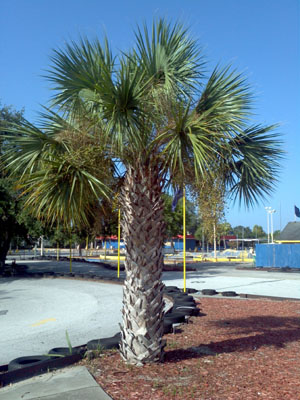The outdoor photograph captures a distinctive short, stubby palm tree characterized by its broad, dark grayish trunk and several green palm fronds growing from the top. The palm tree, approximately 12 to 15 feet tall, is planted in a bed of mulch and is set within what seems to be a racetrack area lined with black tires for protection. To the left, part of the roadway is visible, also bordered with tires, while the surrounding environment features abundant concrete surfaces and structures such as short buildings, a blue wall, and yellow poles. The background reveals a gleaming blue sky, additional greenery, and possibly distant glimpses of a parking lot or marina-like area with boats.